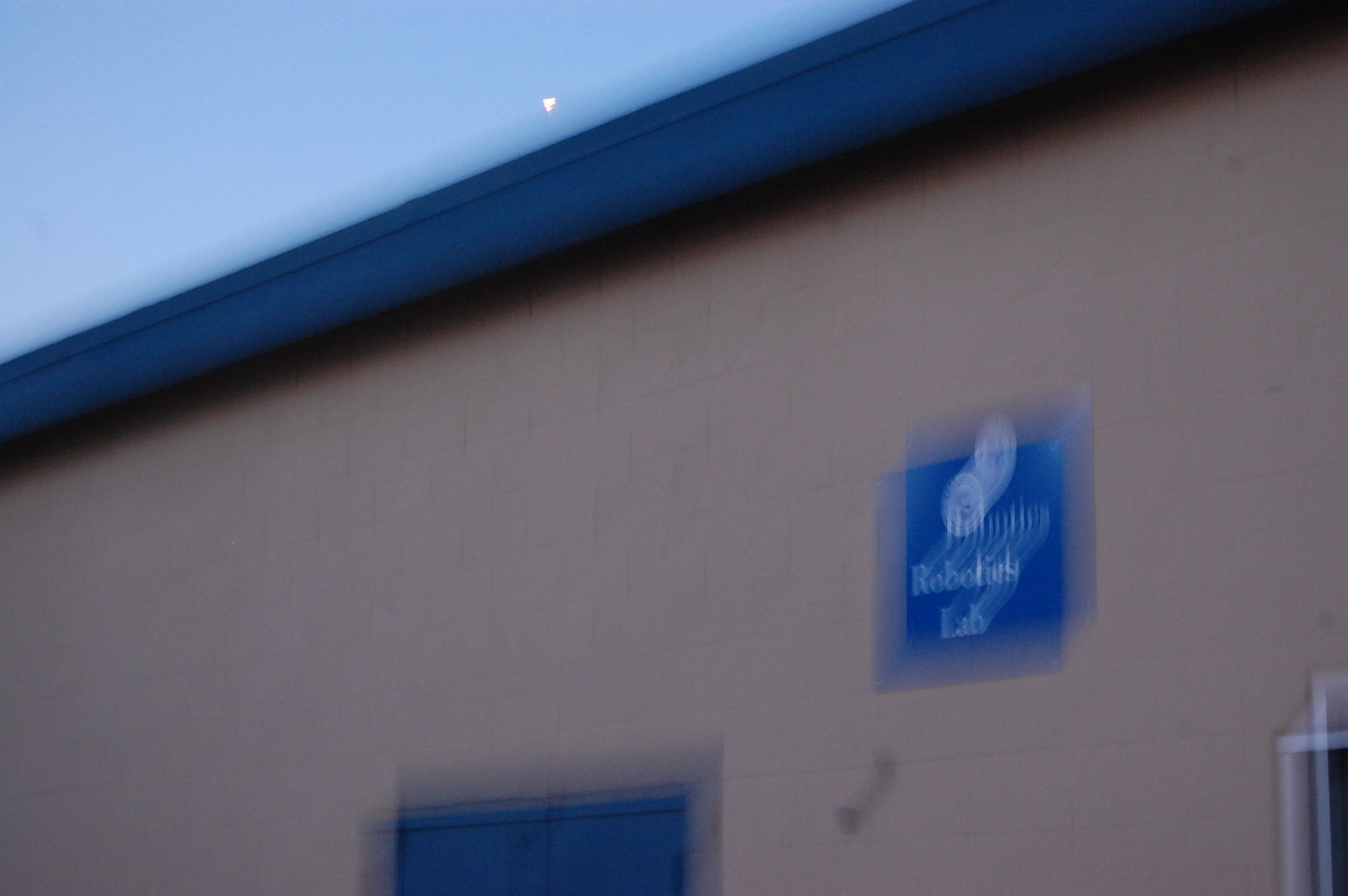This colour photograph, taken during twilight, is characterized by a noticeable blur due to camera movement, resulting in a double ghosting effect on all elements within the image. The scene is set outdoors and hints at a transition towards dusk, indicated by the subdued light and an underexposed appearance.

In the top left corner, a patch of blue sky is visible, while the right diagonal of the frame is dominated by a light brownish-beige brick building. The building's outline ascends diagonally, drawing attention upwards. Affixed to the side of this structure is a sign, challenging to decipher due to the motion blur, but it clearly contains the word "Lab" as part of its text, suggesting that the building houses some kind of laboratory.

Architectural details such as the roofline are evident, and the image also partially captures a set of double doors at the bottom, which, like the sign, are a dark blue. This colour is consistent across various features of the building, likely indicating the brand's chosen palette. Despite the blurriness, the photograph conveys the contrasting textures and hues, subtly hinting at the building's purpose and visual identity.